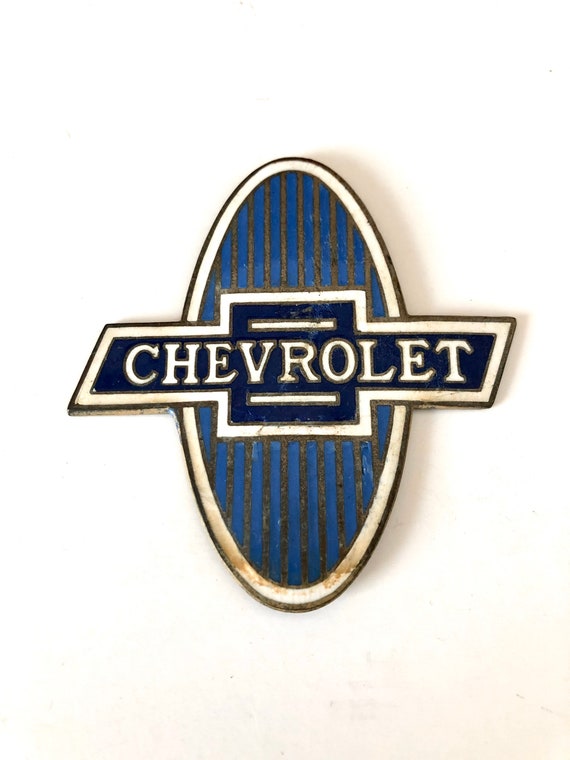The image features a vintage Chevrolet logo set against an off-white, eggshell background. The logo is oval-shaped and prominently displays the word "Chevrolet" in white capital letters spanning horizontally across the center. The text is flanked by two horizontal white lines, one above and one below. Surrounding the letters is a white border, which is further encircled by a black border. The main body of the logo is filled with blue and black vertical stripes, suggesting a worn or aged appearance. The outermost edge of the oval has a golden border. This intricate insignia, likely from an old automobile, lies flat and features subtle signs of dirt, adding to its vintage character.